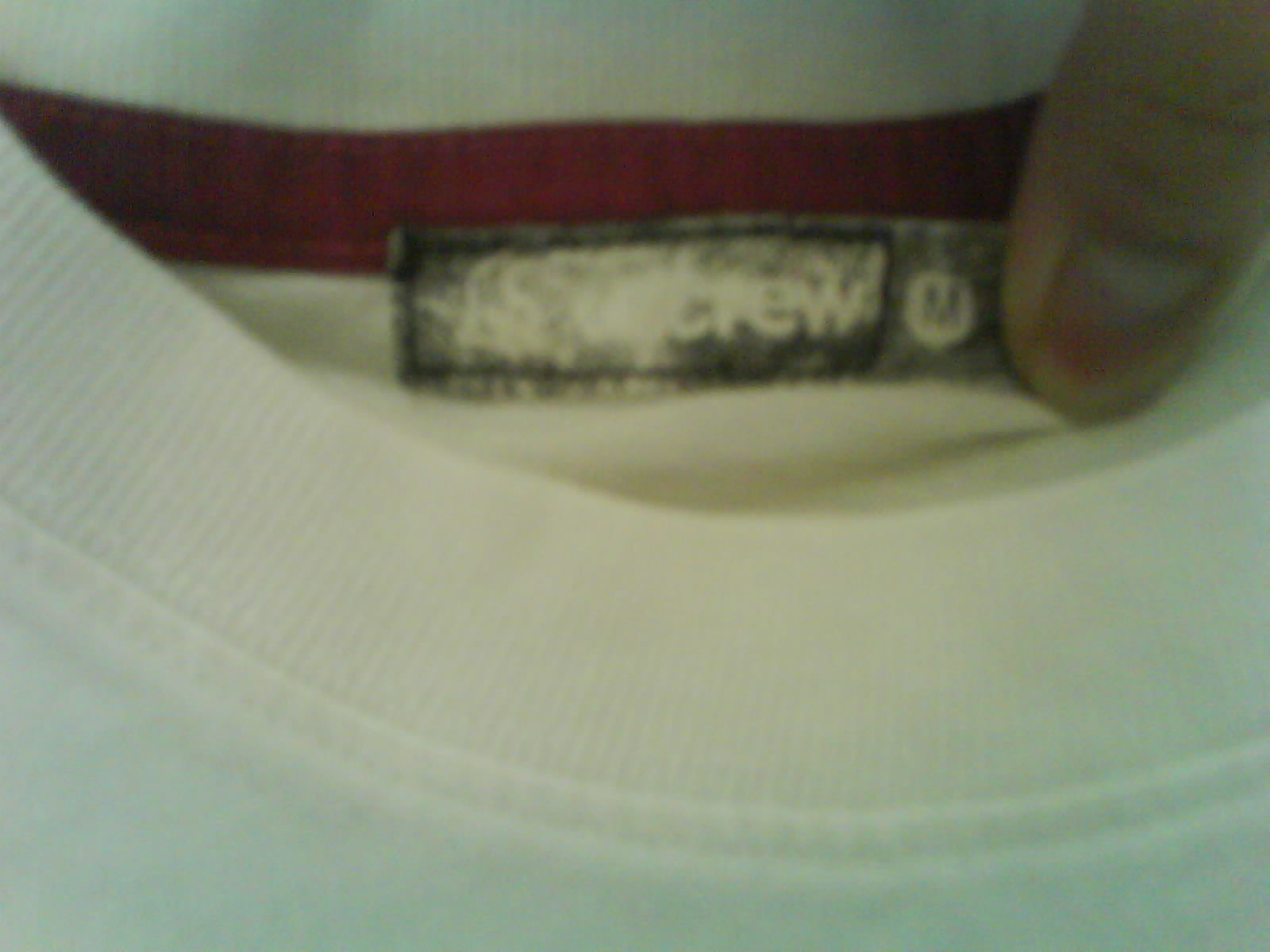The low-quality color photograph, featuring a grainy and slightly washed-out look, captures a close-up of a white crew neck shirt's neckline. The neckline, curved and extending out of the frame, suggests the garment might be a sweatshirt. Prominently visible is a red band running horizontally along the back inside the collar. At the forefront, there’s a worn label displaying partial text, notably the letters "C-R-E-W." To the right, within a gray tag, is a white circle with a black "M," indicating a medium size. A thumb, possibly female due to the nail shape, is placed near the label, with the fingernail pointing downward, providing a sense of scale and orientation.